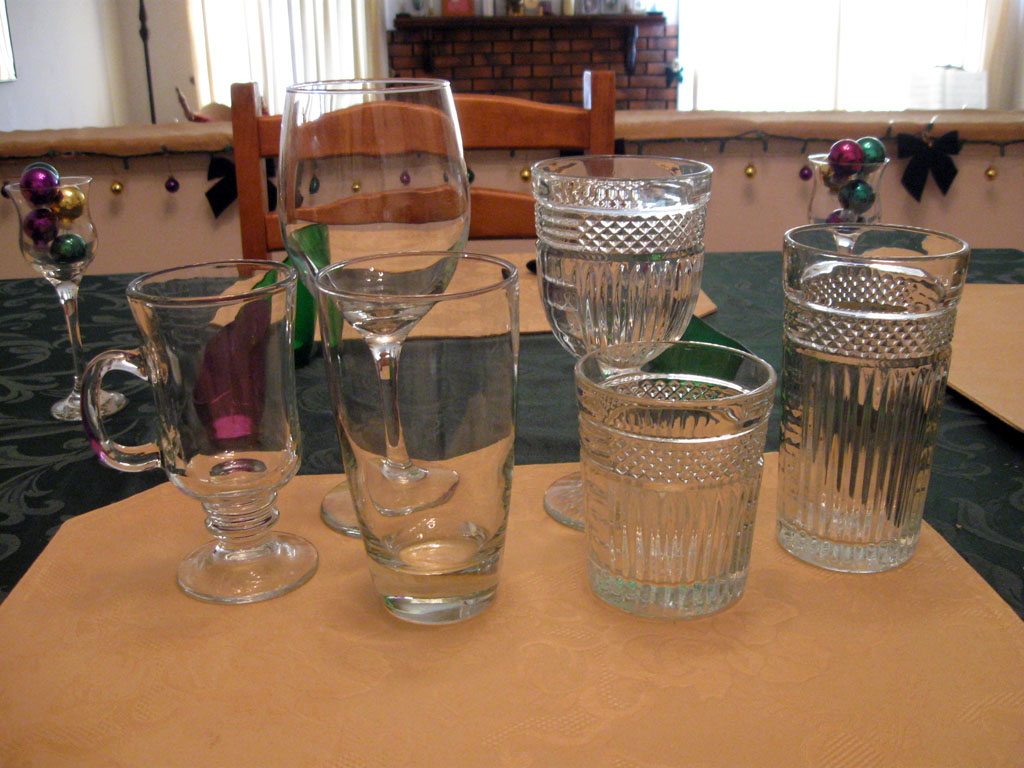The image portrays a collection of varied glasses arranged on a table with three visible brown placemats, which have an indistinct, possibly floral pattern. The glasses are diverse in design: the leftmost is a goblet-shaped glass with a handle, adjacent to a classic wine glass. In front of the wine glass sits a standard beer glass. Further to the right and slightly behind is an ornate goblet with a diamond hatch design. In the foreground, there is a shorter, similarly patterned glass and a full-sized cylindrical glass with vertical ridges. Notably, two wine glasses with decorative orbs resembling Christmas ornaments, in purple, yellow, and green hues, are also present. A brown wooden chair and a length of unlit Christmas lights are visible in the background, along with additional similar ornaments. Beyond the table lies a wooden counter and a small brick structure topped with books, flanked by two bright windows with curtains.